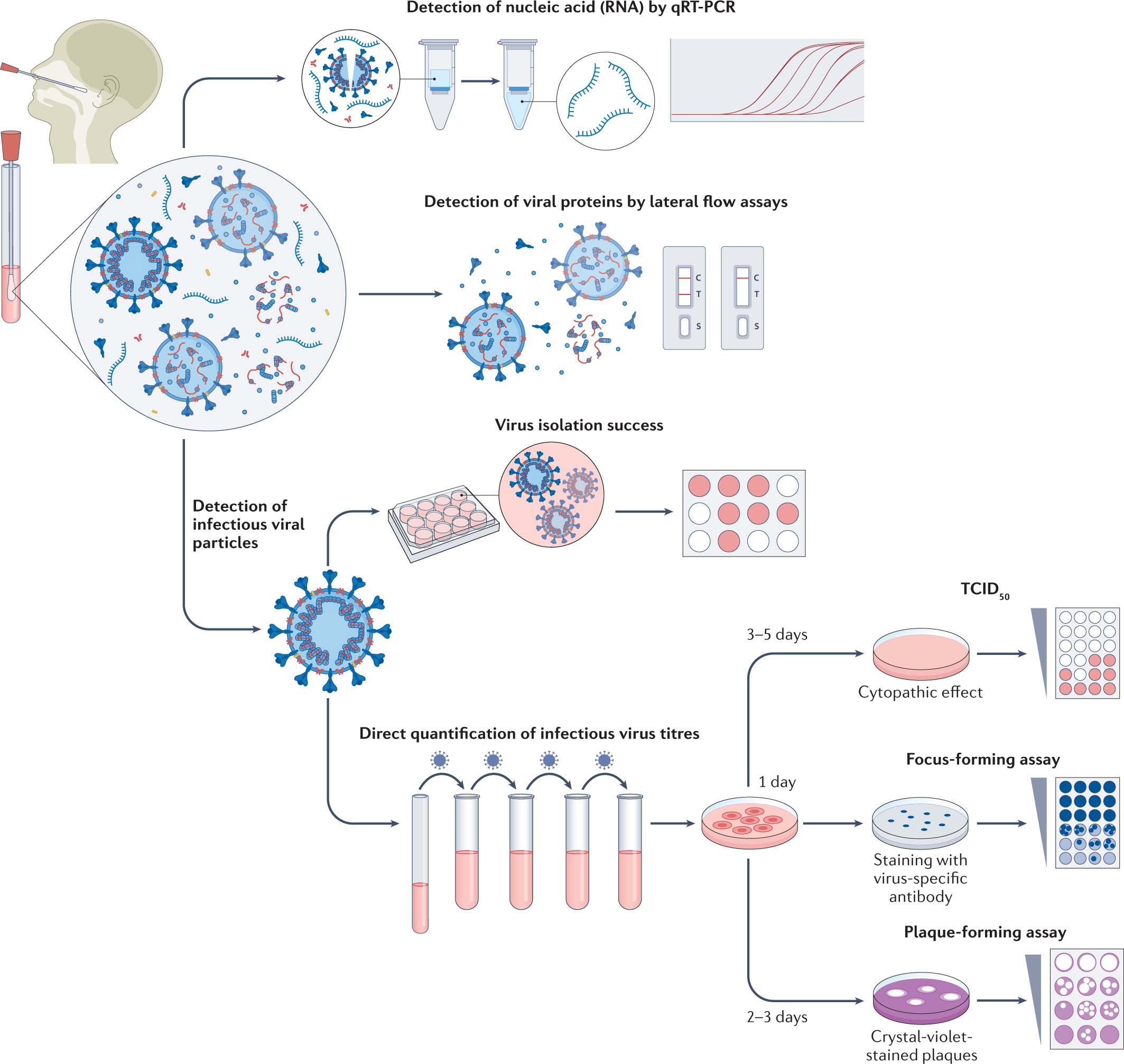This illustration is a detailed, step-by-step instructional diagram depicting the detection of nucleic RNA by QRT-PCR. It employs clean, minimal colors for clarity and ease of understanding. The process starts on the left, illustrating a person with a nasal swab being inserted. Following this, the swab, now potentially containing viral particles, is placed in a test tube. The depiction continues with the test tube’s liquid contents, showing the subsequent detection of viral RNA.

Next, the workflow diagram highlights the detection of viral proteins via lateral flow assays, with images showcasing the viral particles. Moving further, it illustrates the isolation of infectious viral particles and their transfer to petri dishes for further testing. There is an indication of the isolation process showing detailed circular trays where the particles are identified.

Arrows guide you through the diagram, showing additional test tubes and examples of time-sensitive testing over several days. This includes various levels of cytopathic effects and staining of virus-specific antibodies in petri dishes, depicted with the use of crystal violet plaques. The diagram is meticulous in its representation, with each step clearly marked, making the entire RNA detection process coherent and comprehensive.